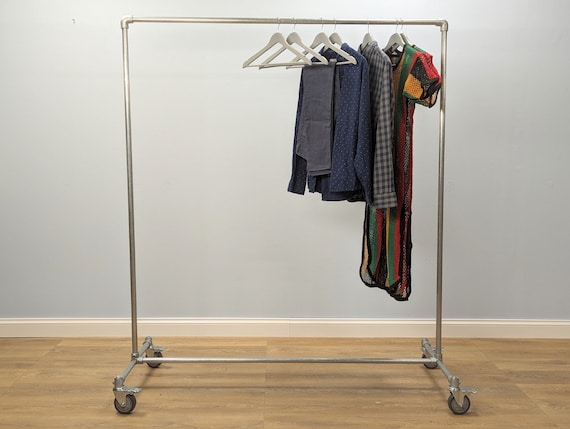The photograph features a portable, industrial-style clothing rack constructed from silver metal pipes, complete with pipe fittings and heavy-duty caster wheels that include locks for stability. The pipe frame, which has a rectangular shape, stands on a light-colored wooden floor in front of a light gray wall adorned with a cream-colored mop board. Among the wooden hangers on the rack, two or three are empty, while the remaining ones display a variety of garments. These include a pair of slacks or jeans, a dark sports shirt, a blue and white polka dot shirt, a blue and white plaid shirt, and two multicolored robes or mesh dresses featuring shades of yellow, green, red, and black. The overall design of the clothing rack is utilitarian and functional, accentuated by its substantial and industrial aesthetic.